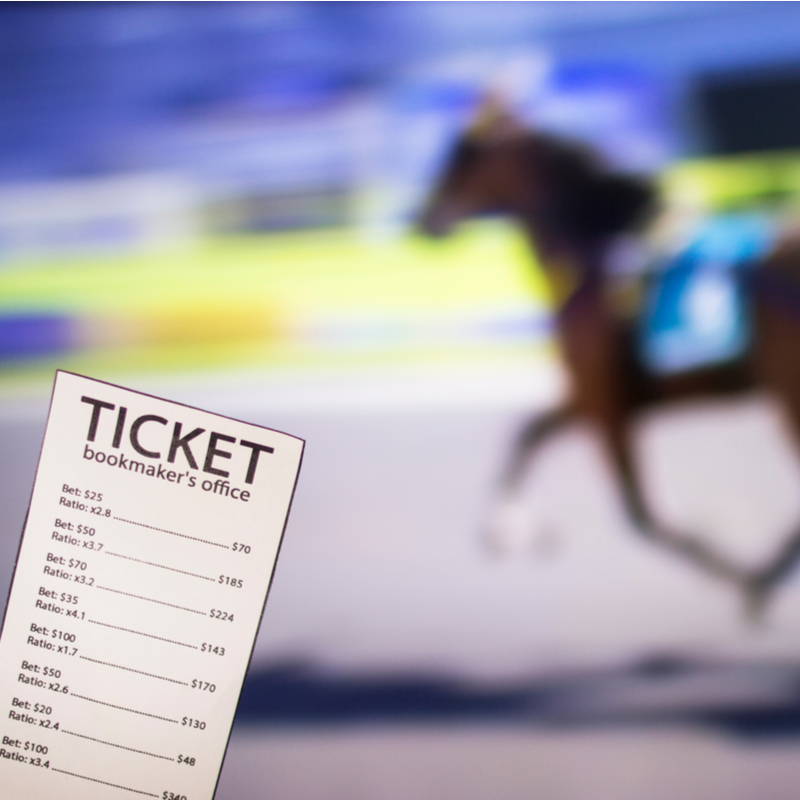The image showcases a highly blurred and out-of-focus scene, which appears to depict a dark brown horse with a blue saddle running on an outdoor horse racing track, evidenced by the blue and yellow hues in the background and a shadowy white ground. Prominently featured in the bottom left corner, there is a sharp, clearly visible rectangular ticket stub resembling a receipt. The ticket stub, marked with "Ticket Bookmaker's Office," lists various betting amounts and their corresponding payouts: bet $25, win $70 at a ratio of 2.8; bet $50, win $185 at a ratio of 3.7; bet $70, win $224 at a ratio of 3.2; bet $35, win $143 at a ratio of 4.1; bet $100, win $170 at a ratio of 1.7; bet $50, win $130 at a ratio of 2.6; bet $20, win $48 at a ratio of 2.4; and bet $100, win $340 at a ratio of 3.4. The juxtaposition of the clear ticket stub against the blurry racetrack scene highlights the betting stakes typically associated with horse racing events.